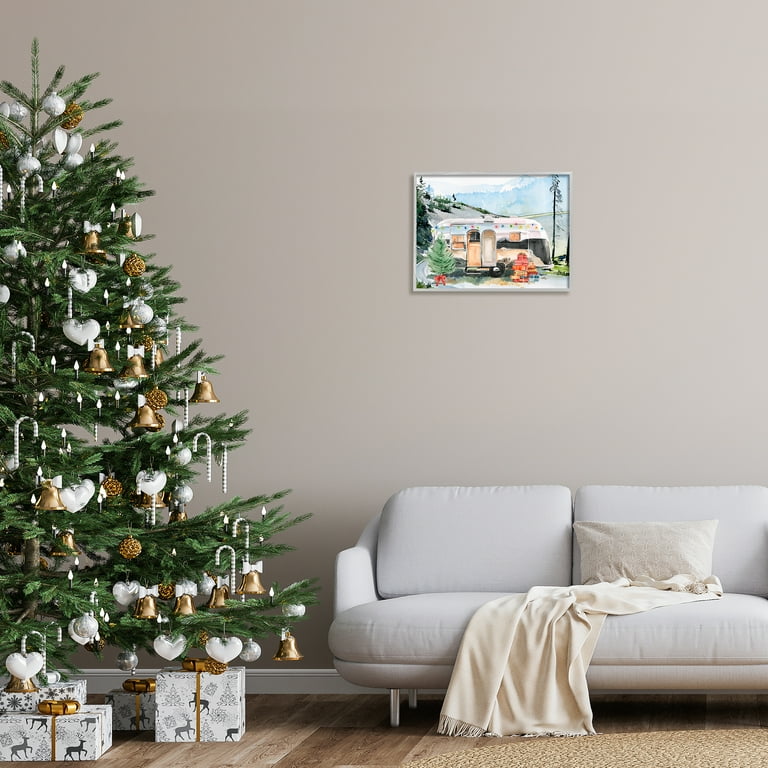In this detailed photograph of a cozy living room, the focal point is a beautifully decorated Christmas tree situated on the left side of the room. The tree, mostly green, is adorned with a variety of festive ornaments, including golden and silver bells, candy canes, heart-shaped decorations, pine cones, and orbs in both silver and gold. Beneath the tree, intricately wrapped gifts in gray and white paper, featuring reindeer designs and topped with gold bows, are positioned. On the right side of the room, there is a plush, white sofa complemented by a cream-colored blanket and an off-white pillow. The back wall, painted a subtle grey, holds a small, rectangular painting above the sofa—a depiction of a camper with Christmas decorations around it. The floor is a warm, brown wood, partially covered by a brown rug in the lower right corner of the image. The overall scene is a harmonious blend of festive charm and cozy, homey elements.